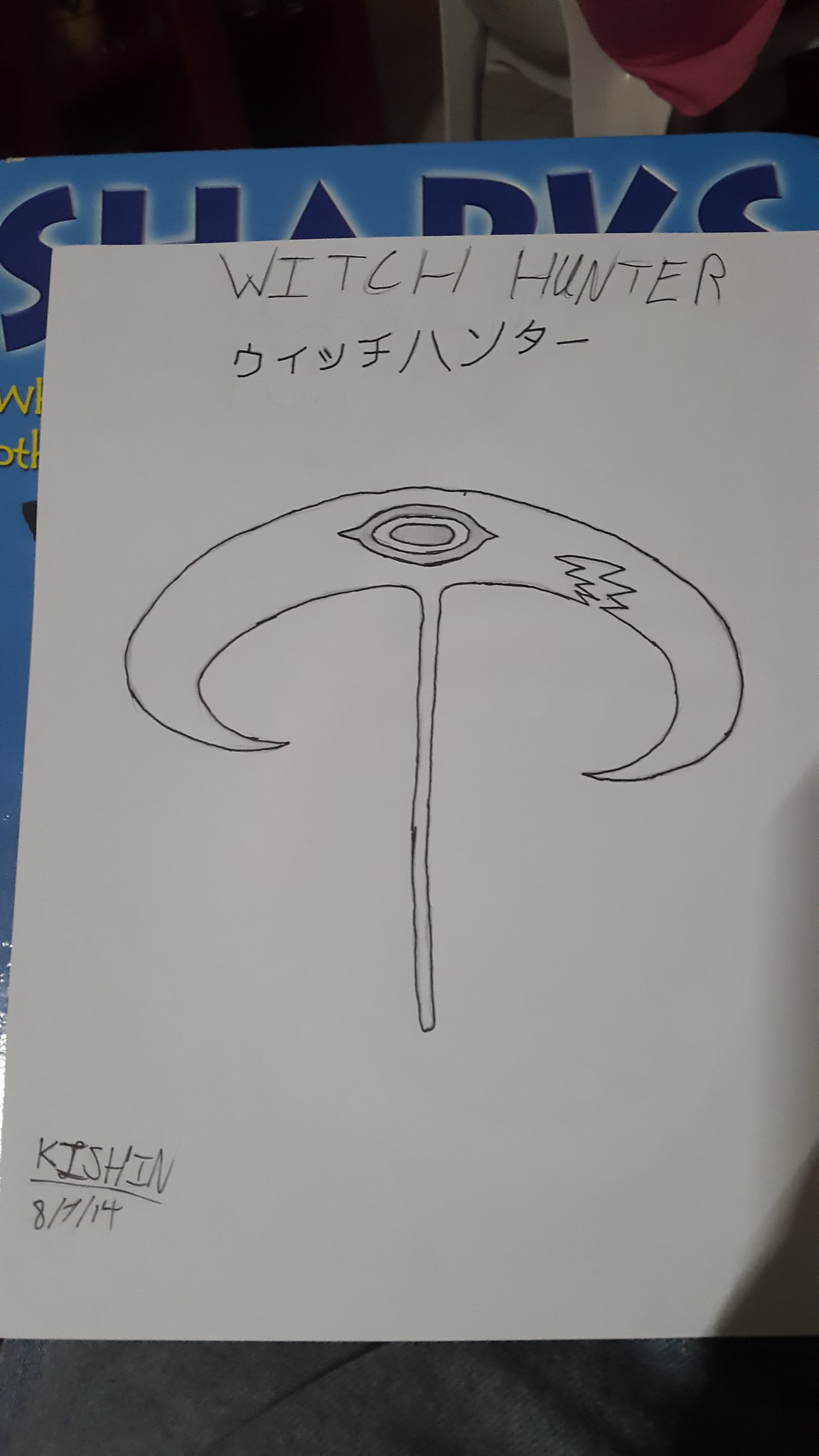This is a highly detailed photo of a vertical sketch rendered in black ink on white paper. The central subject of the artwork resembles a double-edged knife with a curved, ornamental design. The dual blades, which come to a point facing each other within a semi-circle, feature an eye-like figure at their midpoint. Artistically integrated into one of the blades is a striking lightning bolt motif. The handle of this unique weapon is notably thin and appears somewhat crudely drawn, suggesting that it is not the primary focus of the sketch. At the top of the sketch, the words "Witch Hunter" are inscribed, followed by some characters that appear to be in the South Korean alphabet. The artist, who signed the sketch as "Kishin" on the bottom left corner, dated the piece "8-7-14." The background reveals that the sketch is affixed to a poster that features the word "SHARKS" in dark blue, along with partially obscured yellow text. The backdrop appears to be a gray surface, likely flooring or wall material.